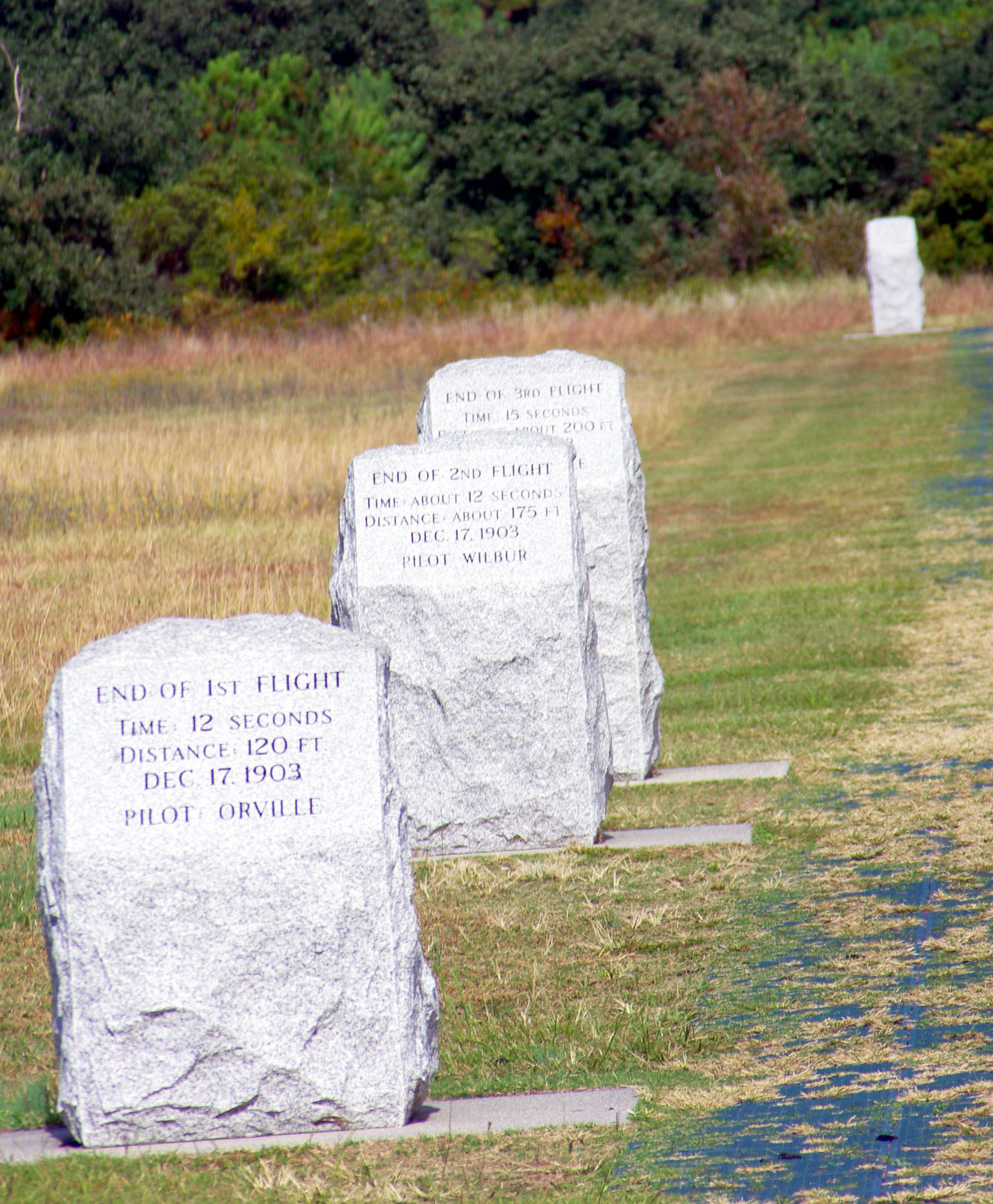In this photograph, we see a grassy area of a cemetery-like setting, marked by four headstones that serve as historical markers rather than graves. The well-maintained grass stretches to the back of the image, interspersed with patches of taller, brownish, and reddish grass. To the left, there's a concrete path or street covered in leaves. Three headstones are prominently aligned in the foreground, resting on concrete slabs, while the fourth stands further back on the right side, its details unreadable due to distance.

The inscriptions on the headstones commemorate the Wright brothers' pioneering flights on December 17, 1903. The closest marker reads, "End of first flight, Time: 12 seconds, Distance: 120 feet, December 17, 1903, Pilot: Orville." The adjacent headstone states, "End of second flight, Time: about 12 seconds, Distance: about 175 feet, December 17, 1903, Pilot: Wilbur." The third marker, partially obscured by the preceding stones, records, "End of third flight, Time: 15 seconds, Distance: about 200 feet." These details highlight this location as the historical site of the Wright brothers' first successful powered flights, with the markers acting as memorials to their revolutionary achievements.